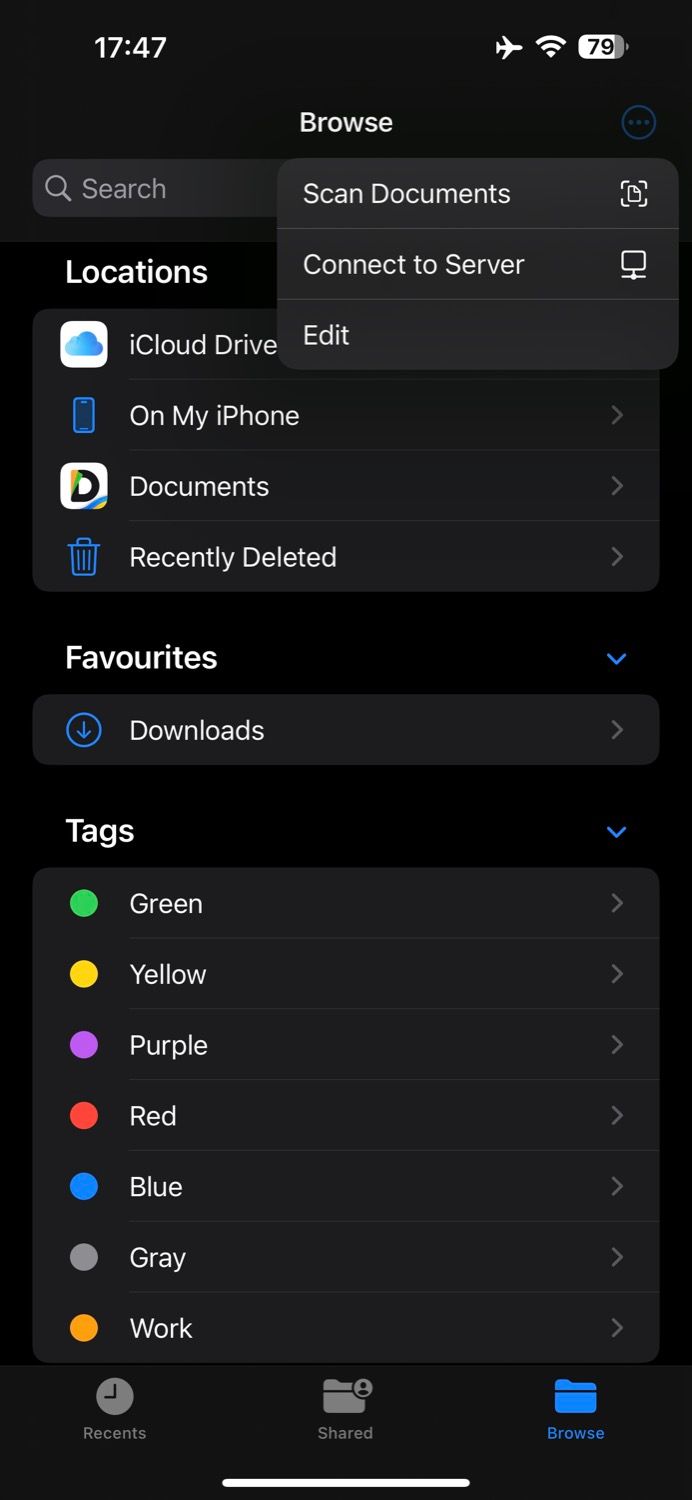The image is a detailed screenshot of an Apple application, though the specific app remains unidentified. At the top left corner, it shows the time the screenshot was taken, which is 17:47 (5:47 PM). On the right side of the top bar, there are three icons: an airplane mode icon, a Wi-Fi icon, and a battery icon displaying 79% charge.

Below this top bar is a navigation section labeled "Browse". Next to it on the right side, there is a small pop-up menu with options that include "Scan Documents," "Connect to Server," and "Edit."

Further down the screen, there is a section titled "Locations" with several options listed:
- iCloud Drive
- On My iPhone
- Documents
- Recently Deleted

Following this is another section named "Favorites," which lists "Downloads." 

The last section is "Tags," displaying colored tags named:
- Green
- Yellow
- Purple
- Red
- Blue
- Gray
- Work (Orange)

Each of these tags has its corresponding color next to the label. This structured layout and labeling system improves the organization and accessibility of the user’s files and resources.